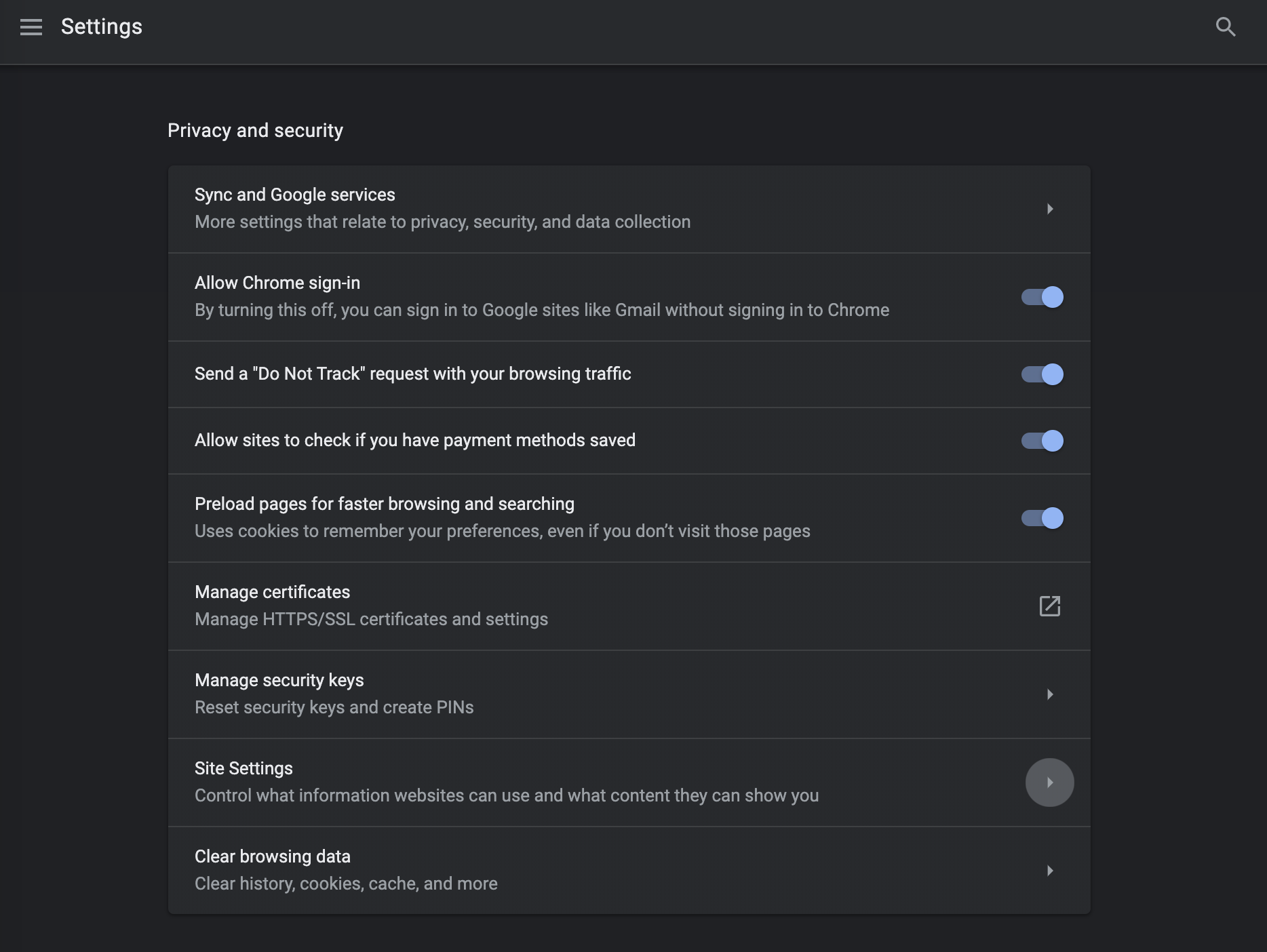The image is a screenshot of the "Privacy and Security" settings page from a computer interface, specifically from a web browser with a dark theme. The top-left corner is completely black, featuring three horizontal lines to represent a menu. To the immediate right of these lines, the word "Settings" appears in white font. In the upper right corner of the screen, there is an icon of a magnifying glass suggesting a search function.

Just out to the right from the left edge, the heading "Privacy and Security" is displayed in white font. Below this heading is a lighter black vertical rectangular area contrasting against the darker black background. Within this rectangle, several settings options are listed, each described with bold white font followed by a more detailed, lighter white font.

1. **Sync and Google services:** 
   - More settings that relate to privacy, security, and data collection.

2. **Allow Chrome sign-in:**
   - By turning this off, you can sign into Google sites like Gmail without signing into Chrome.

3. **Send a 'Do Not Track' request with your browsing traffic:** 
   - (No additional details provided).

4. **Allow sites to check if you have payment methods saved:**
   - (No additional details provided).

5. **Preload pages for faster browsing and searching:**
   - Uses cookies to remember your preferences even if you don't visit those pages.

6. **Manage certificates:**
   - Manage HTTPS/SSL certificates and settings.

7. **Manage security keys:**
   - Reset security keys and create PINs.

8. **Site settings:**
   - Control what information websites can use and what content they can show you.

9. **Clear browsing data:**
   - Clear history, cookies, cache, and more.

On the right side of this rectangular area, there are clickable toggle buttons corresponding to some of the settings. These toggles are blue, indicating they are enabled for items 2, 3, 4, and 5. Item 1 has a small arrow next to it, suggesting it can be expanded. Item 6 has a download arrow, while items 7, 8, and 9 feature right-facing arrows indicating that more options are available upon clicking.